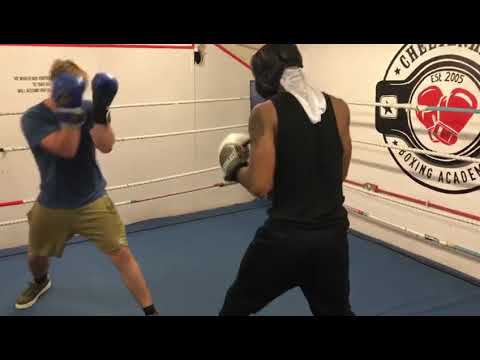In the image, two men are sparring in a blue-floored boxing ring with white lines acting as a fence on the side closest to the wall. The wall on the right side of the image features a prominent logo, which includes a black circle outlined in black with two red boxing gloves at its center, accompanied by the text "Established in 2005" above and "Boxing Academy" below. The man on the left, who has light-colored skin and blonde hair, is wearing a blue t-shirt, mustard short pants, gray sneakers with white soles, and blue boxing gloves. He has his gloved hands up, blocking his face. The man on the right, who has dark skin, wears a black sleeveless t-shirt, black pants, and white boxing gloves. He is also wearing a black padded helmet with a white cloth draping down his neck and partially down his back. The overall color palette of the image includes white, black, red, blue, olive green, brown, and a gold color, contributing to the vivid and dynamic atmosphere of the scene.